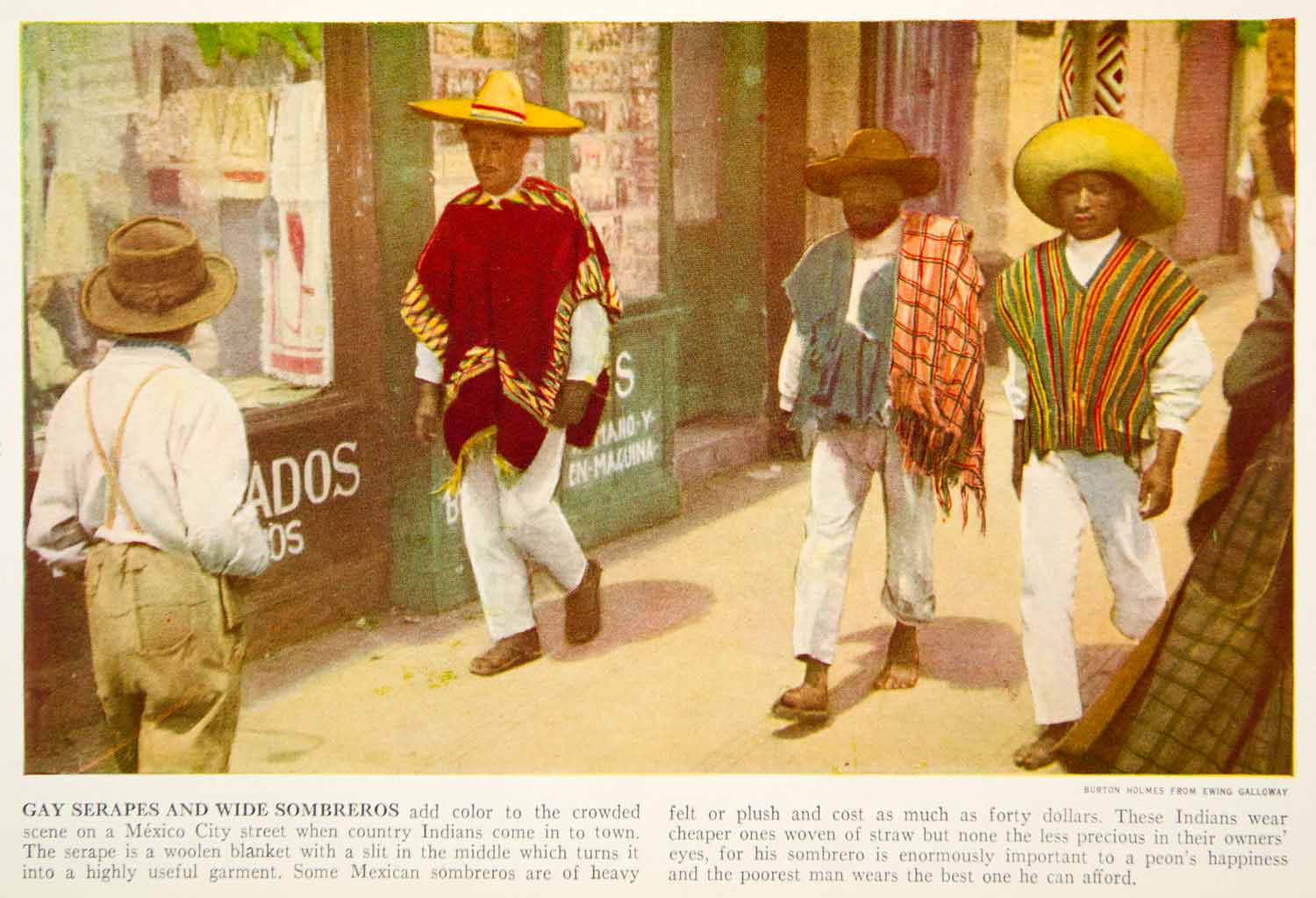In this detailed painting, a bustling Mexico City street scene unfolds, filled with vibrant colors and distinct characters. Four individuals dominate the foreground, all donning traditional Mexican attire. The trio to the left strides purposefully, heading slightly off-center towards the viewer. The leftmost figure wears a striking red poncho adorned with tiger stripes and a large sombrero. Beside him, the central figure sports a smaller dark brown hat, a dark gray serape, and an additional rag draped over his right shoulder. The right figure's poncho displays a vivid mix of green, yellow, and red stripes, capped off with a large sombrero. All three wear white clothing underneath, with the leftmost man resembling a farmer in his white shirt and khaki pants.

In the background, top right, another person appears, seeming to walk away from the scene, while another figure is visible on the bottom left, heading toward the central trio. Storefronts, partially obscured but adding to the street’s lively atmosphere, flank the scene. A storefront sign reads "ados," with more text hidden from view.

Below the image, a caption elucidates the scene: "Gay serapes and wide sombreros add color to the crowded scene on a Mexico City street when country Indians come into town. The serape is a woolen blanket with a slit in the middle which turns it into a highly useful garment. Some Mexican sombreros are of heavy felt or plush and cost as much as $40. These Indians wear cheaper ones woven of straw but nonetheless precious in their owner's eyes, for the sombrero is enormously important to a peon's happiness. The poorest man wears the best one he can afford."